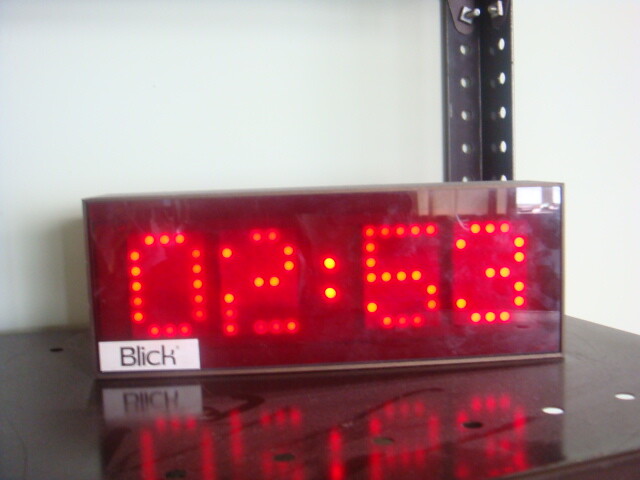This photograph captures a large, older-style digital clock with bright red neon numbers displaying the time "02:53." The clock, branded "Blick," is encased in a glass-like frame that appears to be partially exposed or damaged at the top. Positioned on a black table, the clock casts a reflective red glow onto the table's surface. Behind the clock is a white wall, and to the right, a black metallic post with holes extends down to the table, where sets of screws are visible at the top. The image is illuminated by natural sunlight, highlighting the stark contrasts in the scene.